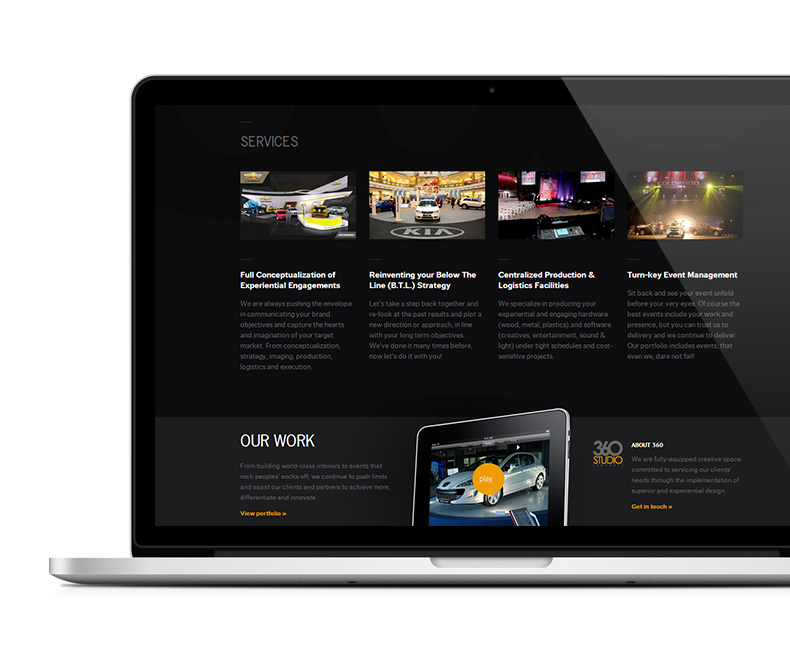A screenshot of a sleek silver MacBook, with the screen displaying a detailed presentation of labeled services encased in a black bezel. The screen highlights several key offerings: 

1. **Conceptualization of Experimental Engagements:** Focused on pushing the envelope in communicating brand objectives to captivate the target market.

2. **Reinventing BTL Strategy:** A collaborative effort to reassess past results and strategize a new direction that aligns with long-term goals.

3. **Centralized Production and Logistics Facilities:** Specializing in the production of experimental hardware using wood, metal, and plastics, as well as creative software for entertainment, sound, and light.

4. **Turnkey Event Management:** Offering comprehensive event management services that allow clients to relax and watch their events flawlessly unfold.

At the bottom of the screen, the text emphasizes the company's continuous effort to push limits, innovate, and assist clients in achieving their goals through world-class interiors and unforgettable events. There are also buttons labeled "View Portfolio" and "Get in Touch," with the latter positioned at the bottom right next to a section about "360 Studio," which is described as a fully equipped creative space dedicated to superior and exponential design. Additionally, there is a play button located at the bottom center of the screen for viewing a video.